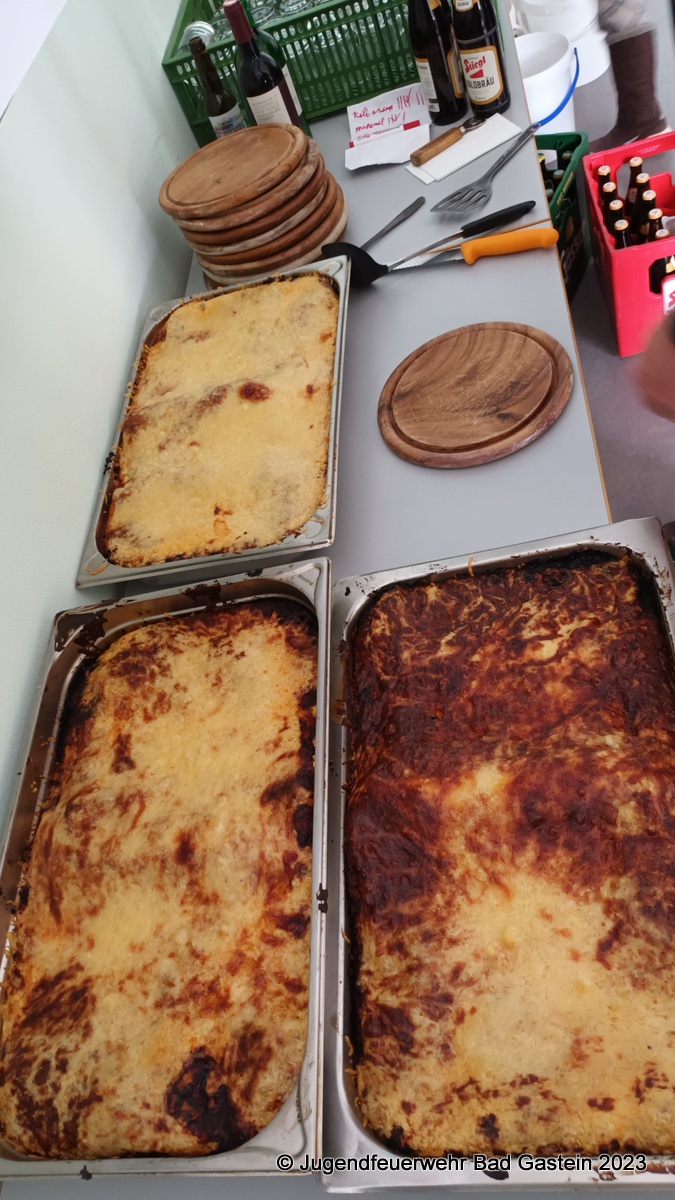This image captures an indoor setting featuring a white countertop laden with three large, rectangular silver pans filled with an ambiguous, cooked dish that resembles either lasagna or enchiladas. The food appears white and dark brown in some areas, with slightly blackened corners. Surrounding the pans is an array of party-related items: a stack of wooden plate-like circles, a pile of spatulas, and a variety of wine and beer bottles. On the white floor in the background sits a red crate filled with more bottles. Text in German, including an unpronounceable name followed by the copyright symbol and the year 2023, is displayed at the bottom of the image. The setting, possibly a kitchen or outdoor patio area, exudes a festive, organized ambiance.